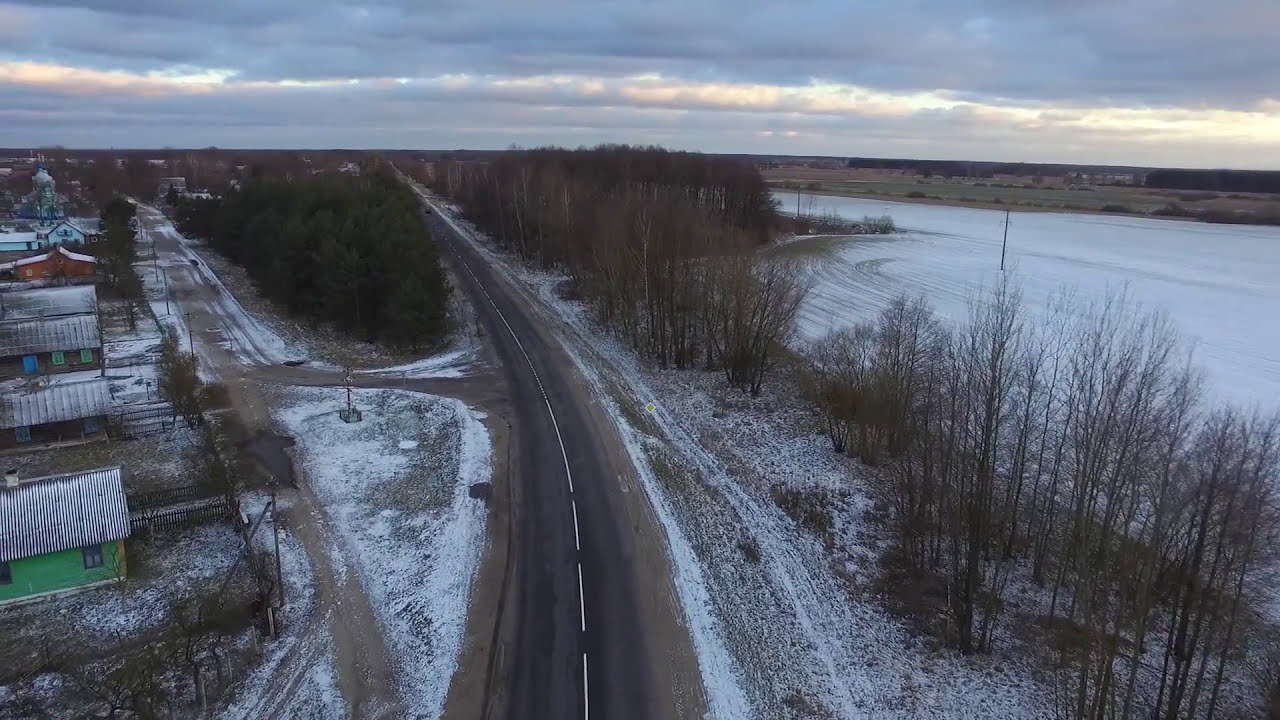The image is an angled high aerial shot, likely taken from a drone hovering approximately 100 feet above a small country road that runs through the center of the photo, slightly veering to the left into the distance. This road, akin to a small country highway, is set within a snowy, wintry landscape typical of small-town America, potentially in the Midwest or Northeast, possibly even Pennsylvania. On the left side of the road, there is an access road leading to several older, worn-down houses in colors such as green, brown, dark red, orange, and light blue, some with corrugated steel roofs lightly dusted with snow. A large green tree can be seen in between the access road and the main road. Further left, the landscape transitions to evergreen trees and more residential buildings, including what might be a small church. To the right of the road is a thin line of leafless trees, beyond which stretches farmland covered with a smattering of snow. In the far background, more buildings are visible. The sky is heavily clouded with just a strip of light breaking through, casting a faint illumination over the serene rural scene.